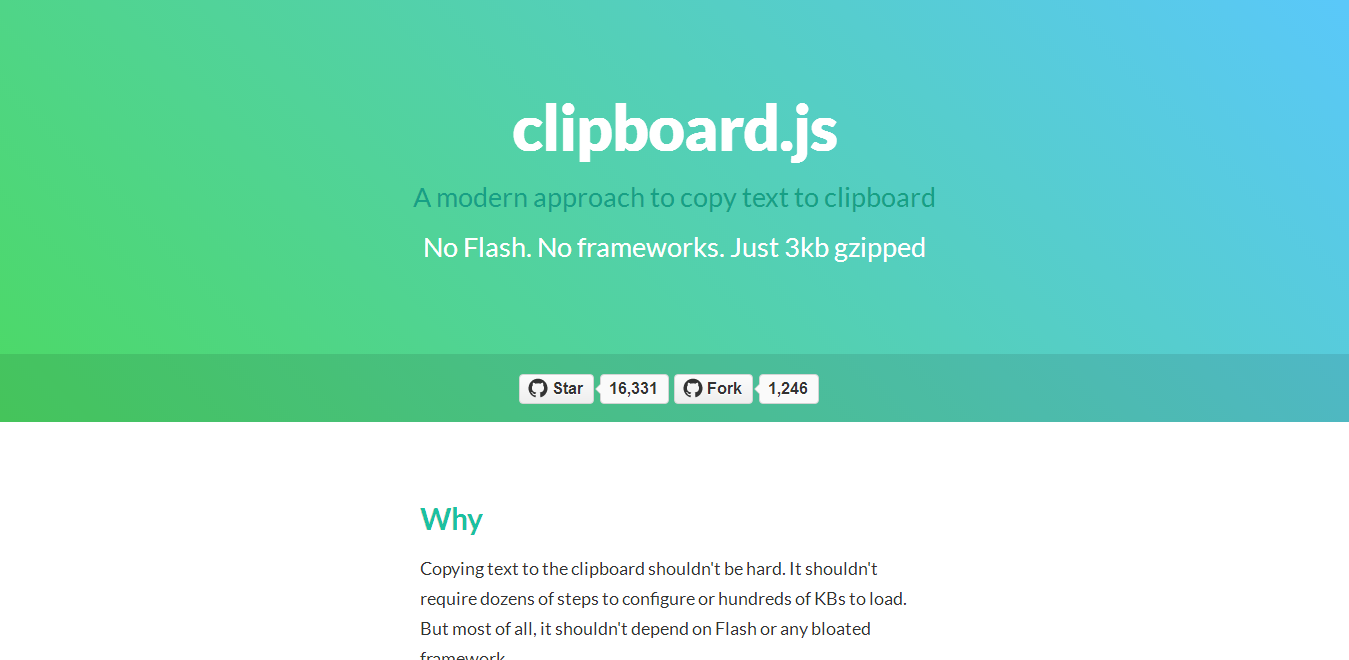This is a detailed screenshot of the Clipboard.js website, a modern tool for copying text to the clipboard without the need for Flash or heavy frameworks, and the entire script is only 3 KB zipped. The website's design features a gradient background that transitions from green to blue in the upper half, while the lower half remains plain white. The green-to-blue gradient section includes key statistics, such as "Star" with the number 16,331 and "Fork" with the number 1,246, indicating the popularity and usage metrics on GitHub. Both sections differentiate text colors, with some text in white, some in black, and some in green. In the white section, the site emphasizes its core value proposition with the statement: "Copying text to clipboard shouldn't be hard. It shouldn't require dozens of steps to configure or hundreds of KB to load. Most importantly, it shouldn't depend on Flash or any bloated framework." This clearly markets Clipboard.js as a lightweight and efficient solution for developers.